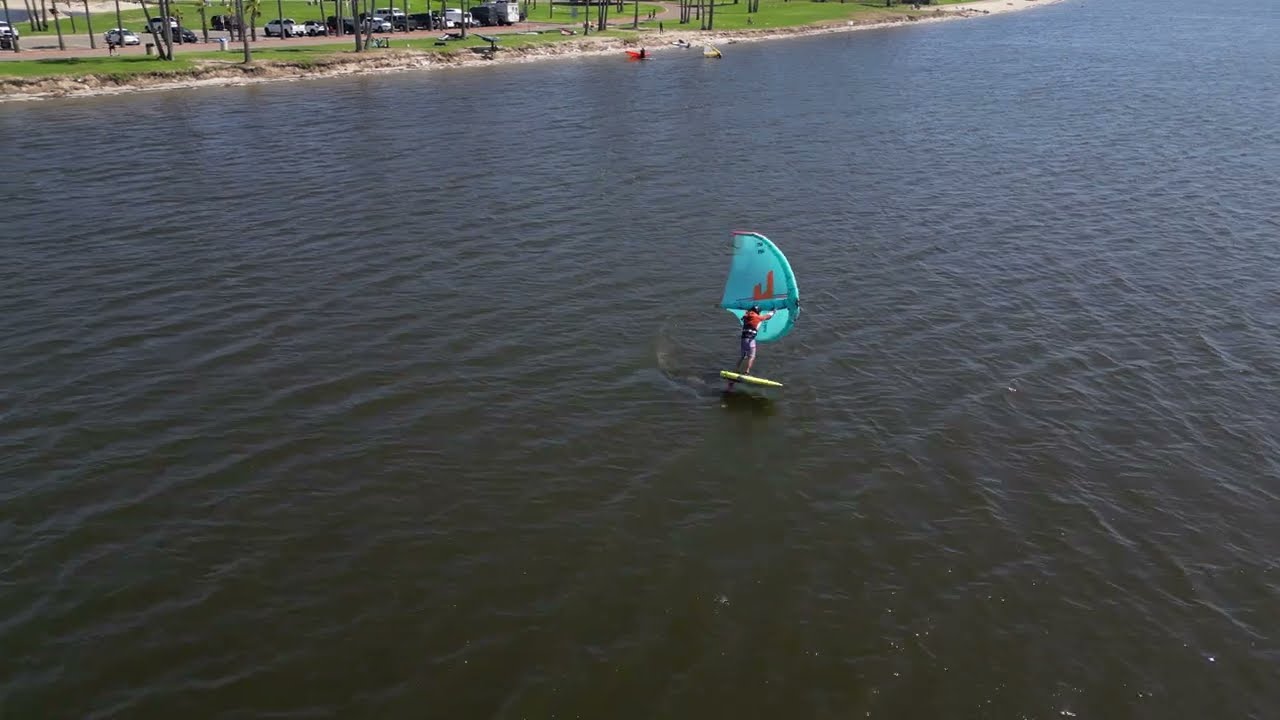A person is windsurfing on a relatively calm body of water, colored a dark blend of blue and green with a few ripples. The person is riding a yellow surfboard and is dressed in a red shirt and light purple pants. They’re holding a light teal sail featuring a red emblem in its center. The sail is primarily flat, rounded on its right side, and has a sharp point aimed downwards towards the water. 

In the background, on the upper left side of the image, you can see the shoreline adorned with green grass and tree trunks without visible leaves. A busy parking lot filled with cars is situated behind the grass, indicating it's a popular area. Close to the water's bank, near the center of the image, two other individuals are observed. One is on a red surfboard and the other on a light-colored board, adding to the lively atmosphere of the scene.